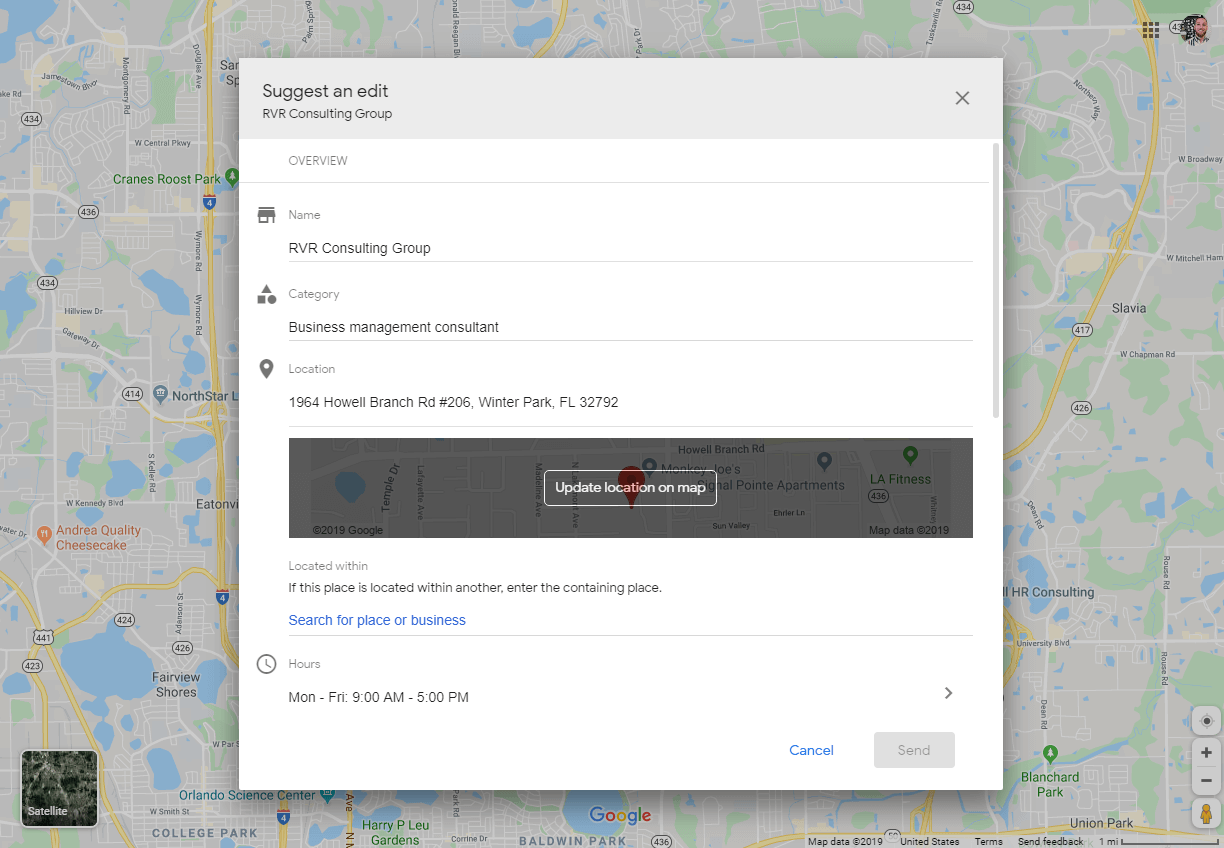This image shows a screenshot of a Google Maps interface. The background features a satellite image of the Orlando area, with notable landmarks labeled such as the Orlando Science Center, College Park, Harry P. Leu Gardens, and Baldwin Park. In the bottom left corner, there's an option to switch to the satellite view. Across the bottom, "Map data 2019 United States" and "Send feedback" are noted.

In the bottom right corner, navigational icons are visible, including a zoom in (+) and zoom out (-) button, and the yellow Pegman icon used for accessing Google Street View. The upper left corner displays additional sections of the map, including Route 434, while the upper right corner reveals the user's personal account information.

A pop-up box in the center of the screen indicates that the user is editing information for "RVR Consulting Group." The top row of the box is gray and reads "Suggest an edit." Beneath this, it says "Overview," with "RVR Consulting Group" listed under the name section and "Business Management Consultant" entered as the category. The location is specified as Winter Park, Florida. The form also allows the user to update their location on the map and includes a field for identifying if the place is within another location. The user added their operating hours. The "Send" button, currently not highlighted, would submit these updates to Google once pressed.